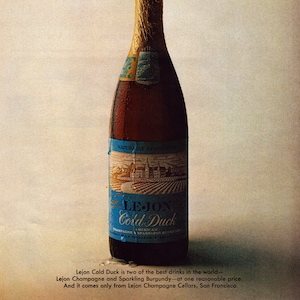The image is an advertisement showcasing a dark brown glass bottle, likely containing wine or beer. The bottle features a blue label adorned with a drawing of a vineyard or chateau, slightly shadowed on the right side. Prominently displayed in dark blue text on the label is "Lejeune", followed by "Cold Duck" in large, white cursive letters. The bottle is topped with a distinctive gold foil wrapper that adds a touch of elegance and sophistication. Beneath the main portion of the label, smaller, fine print provides additional product details, though the text is not easily readable. The backdrop of the photograph is a medium shade of white, ensuring the bottle stands out as the focal point of the image, reflecting a glossy magazine quality.